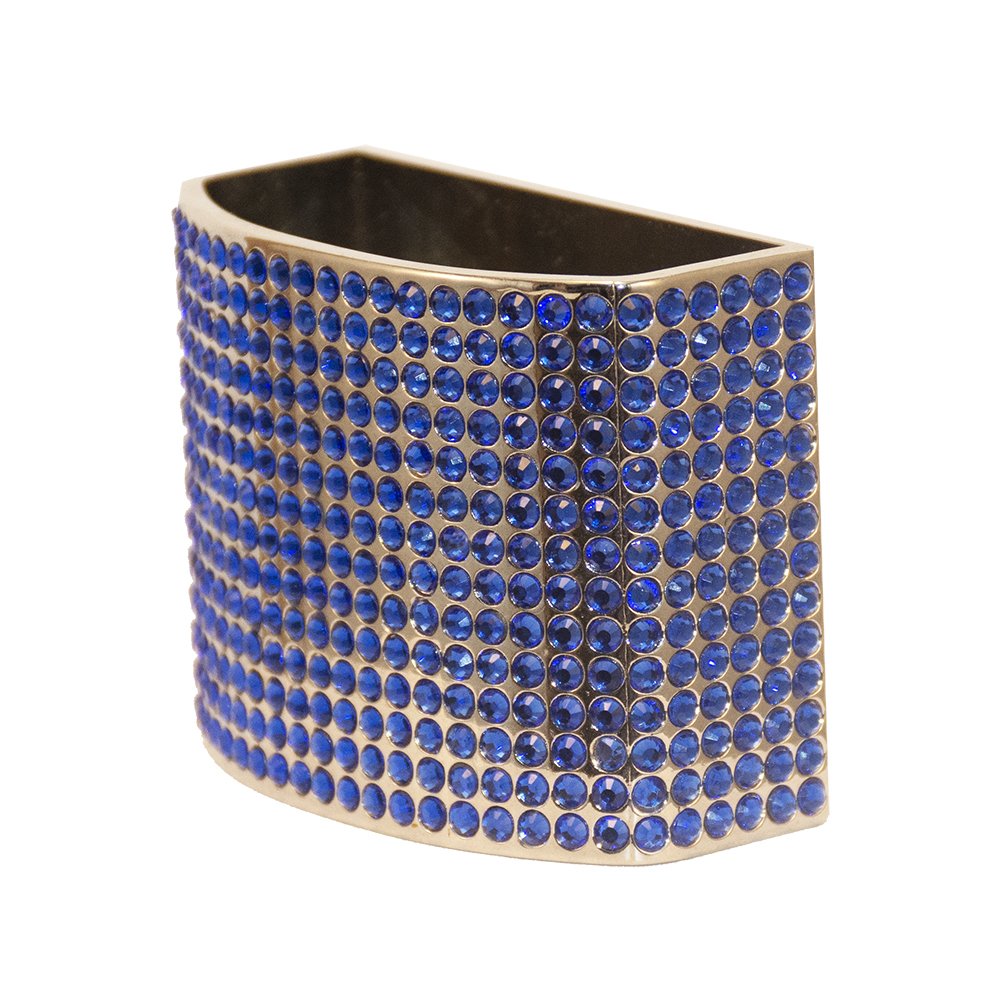The image shows a close-up of a metallic container with a unique shape, reminiscent of a cuboid but with one side slightly curved outward. The container, which may function as a jewelry or toothbrush holder, is adorned with an intricate design of small blue gemstones arranged in symmetrical horizontal rows and columns, with approximately 20 rows in total. These blue circular stones are perfectly embedded into the shiny silver surface, creating a striking contrast and allowing glimpses of the metallic gold base beneath. The container has a flat back and thin walls, with its open top lid revealing a dark grey or black interior. The entire background of the image is a clean, stark white, further highlighting the container's detailed, bedazzled appearance.